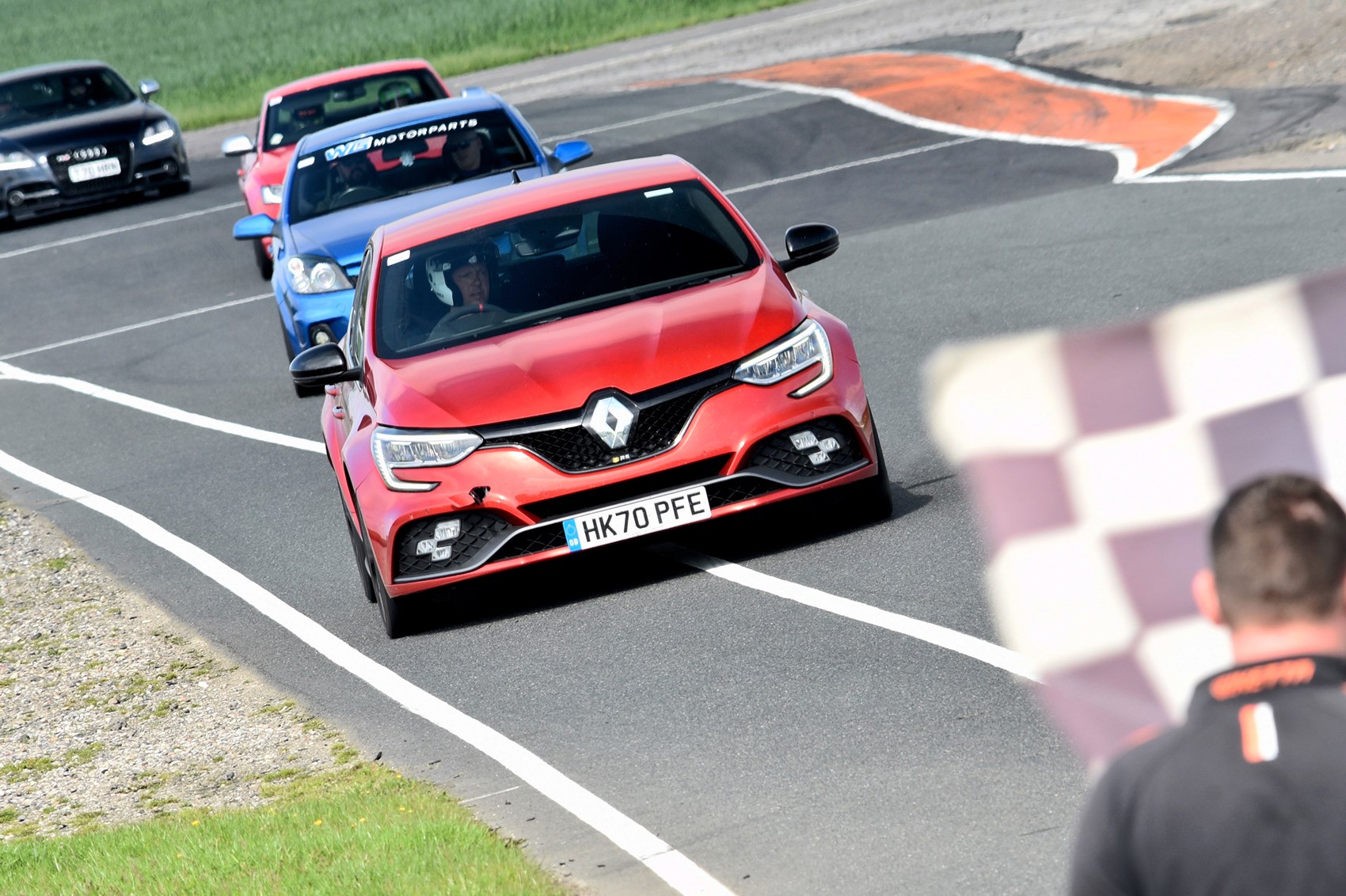The image depicts an intense racing scene featuring four cars on a track. The lineup consists of a red car in the lead, followed closely by a blue car, another red car, and a black car trailing behind. The lead red car carries a license plate reading "HK 70 PFE" and features a distinctive white diamond-shaped emblem on its front. The black car, identified as an Audi by its four-ring emblem, follows at a slight distance. The cars are positioned diagonally on the track with the red and blue cars appearing closer to the viewer and the second red car slightly further ahead. The race takes place on a paved road marked with white lines, surrounded by patches of green grass and dirt. In the bottom right corner of the image, a race official waves a black and white checkered flag, signaling the end of the race.